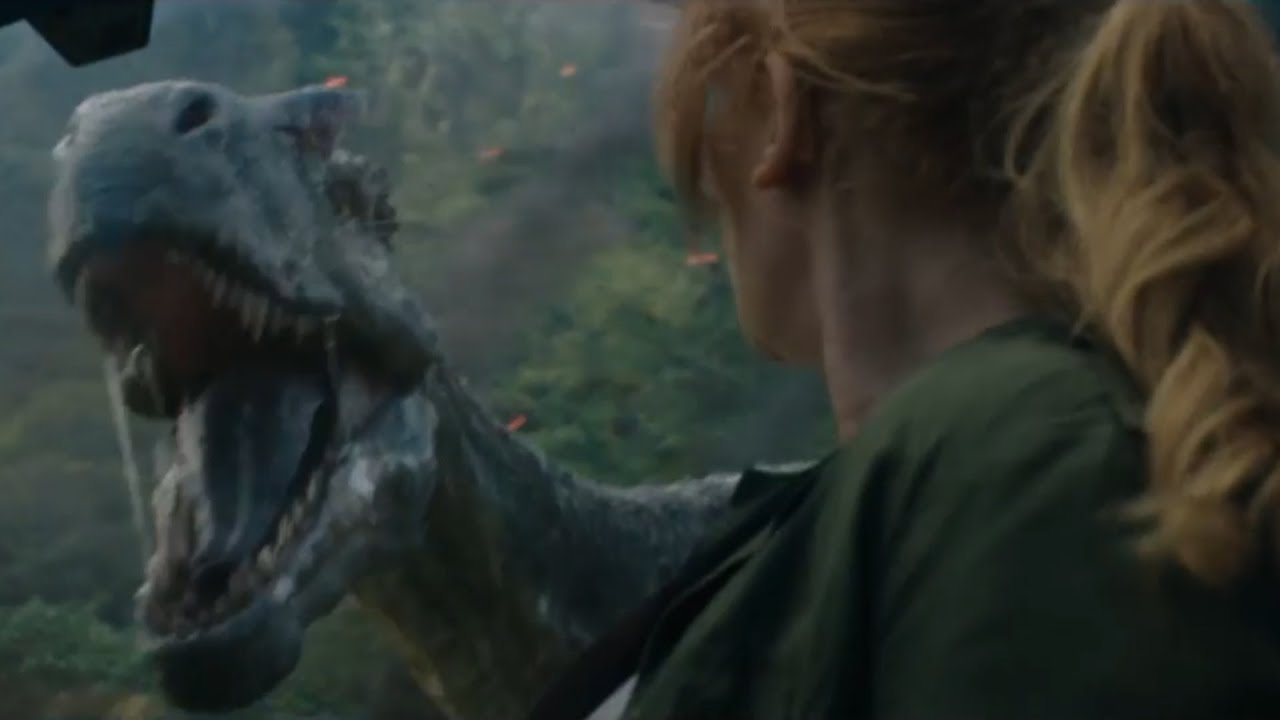The image appears to be a screen capture from either *Jurassic World* or *Jurassic World: Fallen Kingdom*, featuring Bryce Dallas Howard’s character. The setting is a lush, green forest with muted shades and some mountainous terrain, part of which seems to be on fire and emitting smoke. Centered in the foreground is a large, aggressive-looking dinosaur, possibly a T-Rex, with its mouth open, revealing sharp white teeth and a black tongue. Notably, there's a stripe-like mark on the right side of its mouth, possibly saliva. The dinosaur's head is detailed, with visible nostril holes and eye slits, and a long black neck leading down to a glimpse of its body. To the right of this fearsome creature, the side profile of an astonished woman with bulging neck veins can be seen. She has blondish brown hair tied in a ponytail that falls below her shoulder and is wearing a dark green shirt or jacket.